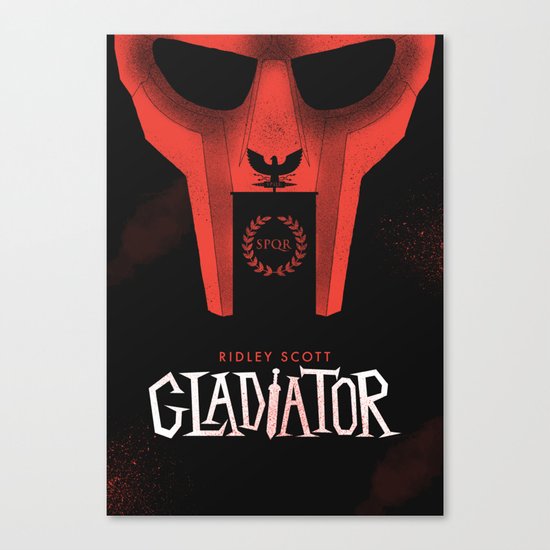The image presents a striking movie poster with a predominantly black background, accentuated by vivid splashes of red reminiscent of blood or paint. Dominating the top half of the poster is an ominous red face mask with dark, unsettling eye holes. Intricately detailed, the nose of the mask features the silhouette of an eagle, while fang-like protrusions are visible from the mask's face. Below the mask, a wreath of leaves or vines frames the letters "SPQR," evoking a connection to ancient Rome. The bottom half of the poster is equally compelling. In stylish red ink, the name "Ridley Scott" is prominently displayed, followed by the intriguing title "Gladiator," where the letter "I" is ingeniously stylized as a sword. The overall presentation of the poster gives it a 3D effect, with shadows at the bottom right and bottom edges making it appear as if it's floating. A light gray border frames the poster, adding to its dramatic visual impact.